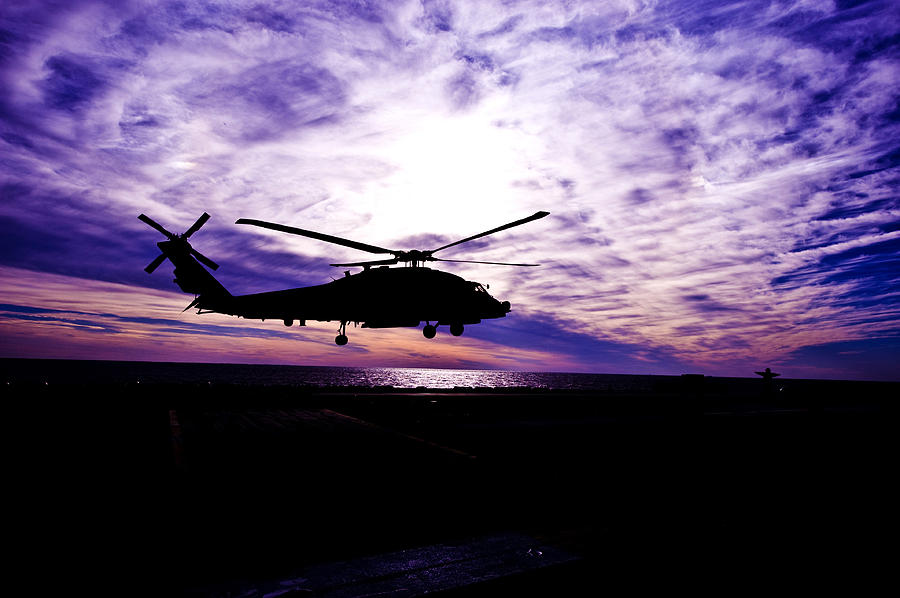In this digitally altered photograph, a helicopter with a four-rotor blade system hovers in silhouette, either landing or taking off against a striking sunset or sunrise backdrop. The sky dominates the upper three-quarters of the image, transitioning from deep indigo and dark purples at the top to warm pinks and oranges along the horizon. Wispy, white clouds are softly illuminated by the setting or rising sun, casting a serene glow. Below the helicopter, calm waters reflect the sunlight, adding a subtle shimmer with visible ripples, contributing to the tranquil atmosphere. The lower part of the image is enveloped in darkness, obscuring details but hinting at a wooden platform or possibly an aircraft carrier deck. A faint outline of an air control tower is discernible in the distance, further suggesting a maritime setting. The overall scene exudes a peaceful yet mysterious ambience, brought to life by the sharp contrast between the silhouetted helicopter and the vividly colored sky.